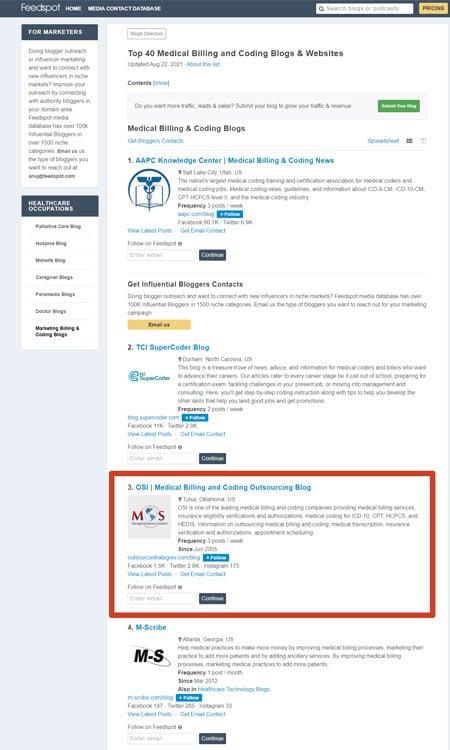The image depicts a webpage from the website Feedspot, indicated by the title prominently displayed. In the top-left corner, navigation options include a home button, a media contact database link, and a pricing button adjacent to a search box positioned at the top-right, enabling users to search for blogs or podcasts. Most of the page's text uses black and blue fonts, though the majority of it—roughly 95%—is blurred and unreadable.

Visible sections include a segment at the left center labeled "For Marketers," followed by an unreadable paragraph. Adjacent to this, another segment titled "Health Care Occupations" lists seven titles, though these are also indiscernible due to the blurriness of the photo. 

Dominating the main body on the right is a header reading "Top 40 Medical Billing and Coding Blogs and Websites." This area includes a context button link, though much of the surrounding text remains blurred and illegible. Beneath, another header states "Medical Billing and Coding Blogs," leading into a list of entries. The first item listed is "1. APC Knowledge Center: Medical Billing and Coding News," accompanied by options to get influential bloggers' contacts and an email contact link. The second item reads "2. TCI Super Coder's Blog." The rest of the text remains obscured and difficult to interpret.